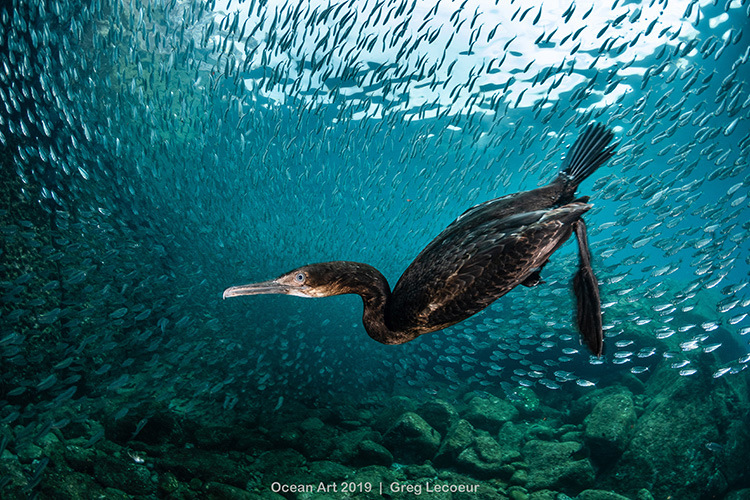This underwater photograph from Ocean Art 2019, captured by Greg Lesseur, showcases a long-billed duck diving beneath the water's surface. The duck, primarily brown in color with a lighter-toned face, has its wings tucked close to its body, revealing one webbed foot and the splay of its tail. The scene is set against a vivid blue backdrop with several gray rocks scattered at the bottom. A large school of tiny fish swarms around the duck, creating a dynamic and lively atmosphere. Contrasting with the predominantly blue surroundings, the surface of the water is visible at the top, with a whitish glow hinting at the sky above.